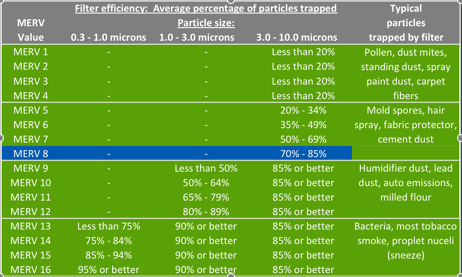The image depicts a detailed screengrab of a color-coded spreadsheet titled "Filter Efficiency: Average Percentage of Particles Trapped," which provides an extensive breakdown of the filtration performance. The top section of the spreadsheet features a gray background with white text, outlining columns for various parameters including NERV value, particle size ranges (0.3-1.0 microns, 1.0-3.0 microns, 3.0-10.0 microns), and "Typical Particles Trapped by Filter." The green background dominates the rest of the spreadsheet, interspersed with white lettering and yellow data points. Each row corresponds to a different NERV value, ranging from NERV 1 to NERV 16, with NERV 8 uniquely highlighted by a blue background. The rightmost column lists various particles, such as dust mites, pollen, sprayed paint dust, mold spores, humidifier dust, lead dust, bacteria, and tobacco smoke, specifying the micron sizes of these particles and the respective filter's trapping efficiency.